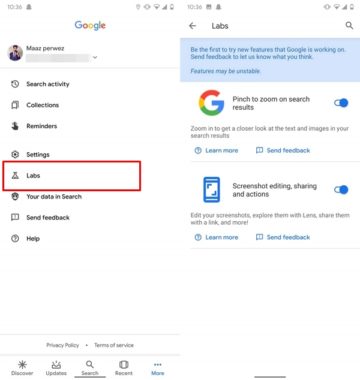This screenshot displays the home screens of two smartphones side by side, both showcasing different sections of Google's interface.

On both phones, the very top left corner shows the current time, and adjacent to it are various status icons including the battery level, Wi-Fi connectivity, and internet status. The phone on the left side additionally displays a Bluetooth icon.

**Left Phone:**
- The center features the Google logo, coupled with a microphone icon.
- Below the logo, there's a gray search bar.
- Toward the left side of this screen, there are eight vertically aligned icons representing different functions.
- Each icon has corresponding text to its right; for instance, the top icon is labeled "Search Activity."
- The fifth icon from the top is highlighted with a red rectangular border, indicating it's selected, and is labeled "Labels."

**Right Phone:**
- This screen shows the interface when "Labels" is selected.
- An arrow pointing left is located at the top left corner, next to the word "Labs".
- A search bar is placed on the right side at the top.
- Below the search bar, there is a blue pop-up message saying, "Be the first to try features in Google," followed by additional information.
- Beneath this pop-up is the Google "G" logo with the phrase "Pinch to zoom on search results" next to it, and it is toggled on.
- Further down, there is detailed information about this feature.
- Following the informational text, there are blue hyperlinks labeled "Learn more" and "Send feedback."
- Finally, at the bottom, there is a section titled "Screenshot editing, sharing and actions," which is toggled on, followed by another line of information below it.